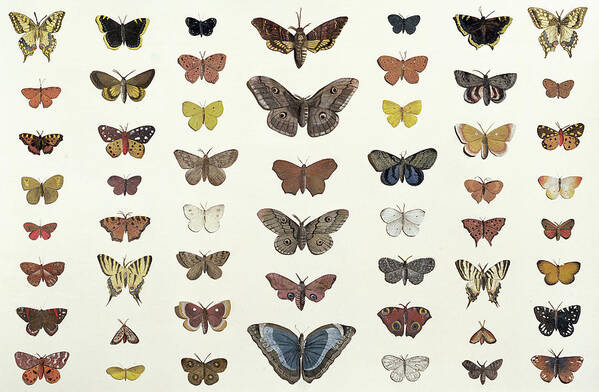The photograph depicts a meticulously arranged collection of butterflies, possibly belonging to an avid lepidopterist. The butterflies, displayed on a white background, are organized into a grid of seven columns and eight rows, making for a very structured and orderly presentation. They vary greatly in size, shape, and color, showcasing an impressive diversity. From tiny black and beige ones to larger specimens with blue, red, yellow, orange, white, and even brown wings with striking blue spots, the array includes earth tones and vivid hues. The larger butterflies predominantly occupy the center row, while the smaller ones are placed towards the outer edges. The clarity of the image is pristine, reflecting bright, well-lit conditions, though it lacks any captions or identifying text that could provide further context about the origins or species of the butterflies.